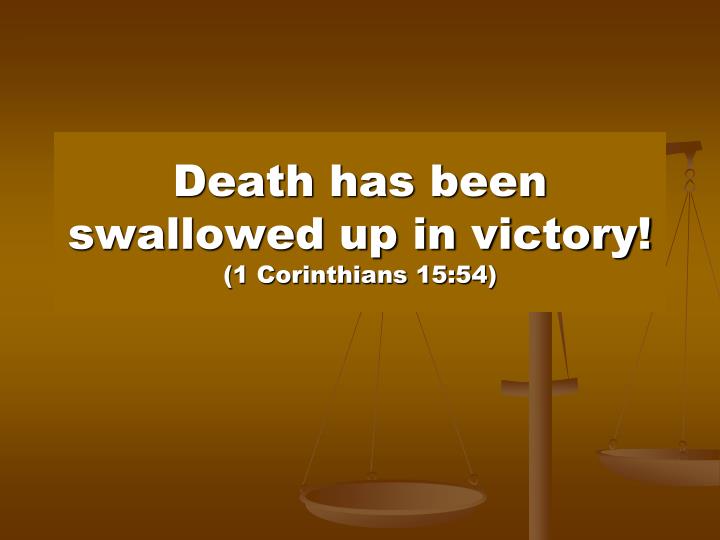The image depicts a biblical quote from 1 Corinthians 15:54, "Death has been swallowed up in victory!" in large white letters. This message is contained within a light brown rectangle situated in the middle of the image. Below the quote, the citation appears in smaller white font within parentheses. Behind this rectangle, a set of balance scales is visible, with the right side higher than the left. Each side of the scale features a circular plate suspended by three strings from a central stand, resembling a traditional depiction of justice scales. The upper part of the image features a darker brown color, transitioning to a lighter brown hue towards the bottom. The entire composition emphasizes the contrast and symbolism of the biblical passage against the background of the scales.